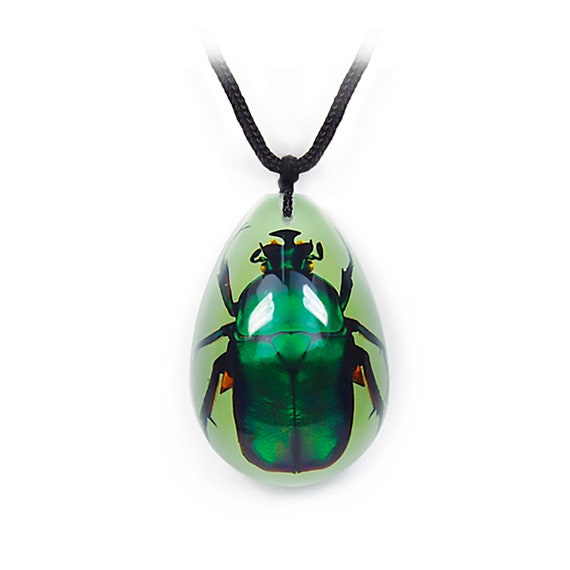This image depicts a teardrop-shaped pendant featuring a green iridescent beetle, encased in a translucent green jewel or crystal. The beetle, which has a high-gloss, dark emerald green shell, exhibits intricate details with six black legs and a green and black head. Additionally, it displays two distinctive orange or red spikes protruding from its back legs. This pendant is attached to a simple black string necklace, with a separate string linking the pendant itself to the main necklace cord. The entire composition is presented against a white background, enhancing the vivid colors of both the beetle and the encasing jewel. The overall appearance suggests a piece meant for display or sale in a jewelry shop, with its high-definition features making the beetle appear almost lifelike.